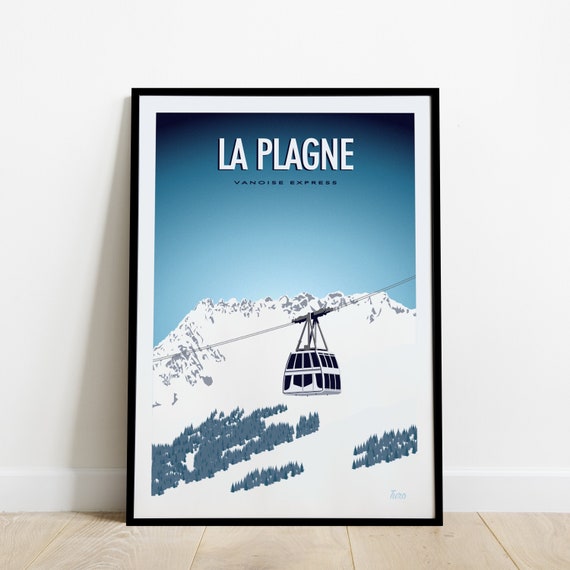The detailed image depicts a framed print propped against a white wall on a light brown wooden floor. The print is framed in black with a white inner border. At the top of the image, large white text reads "La Plagne," followed by slightly smaller text that reads "Vendice Express." The scene within the print shows a snowy, rocky mountain with patches of trees, viewed against a blue sky that darkens towards the corners. A large enclosed ski lift gondola is central to the image, suspended on a cable above the mountainside. The overall artwork maintains a simple yet striking composition.